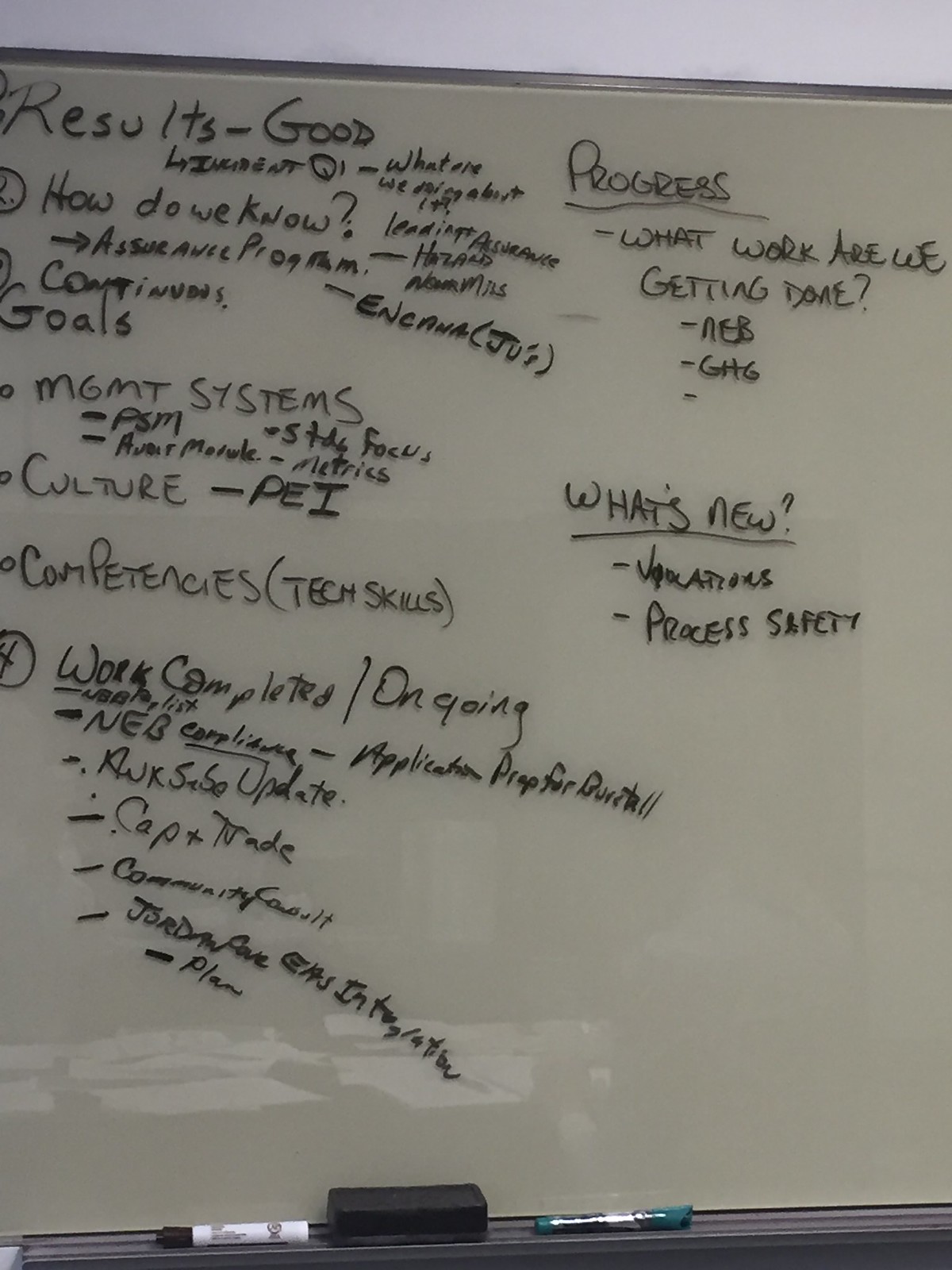The image depicts a somewhat reflective, shiny whiteboard mounted on a wall, photographed at a slight angle. The board is populated with various sections of handwritten text, primarily occupying the left side and top half of the right side, leaving the lower right portion largely empty. The writing is organized into lists with underlined titles, including "results good," "what are," "how do we know," "goals," "management systems," "culture PEI," "progress," "what work are we getting done," "what's new," "vacations," "process safety," "work completed/ongoing," "NEB compliance," and "application prep for something." The handwriting is notably messy. Reflective elements of the board reveal a desk with scattered papers and a faint image of a person seated. At the bottom of the whiteboard, there's a small tray holding a black marker, a green marker, and an eraser between them.